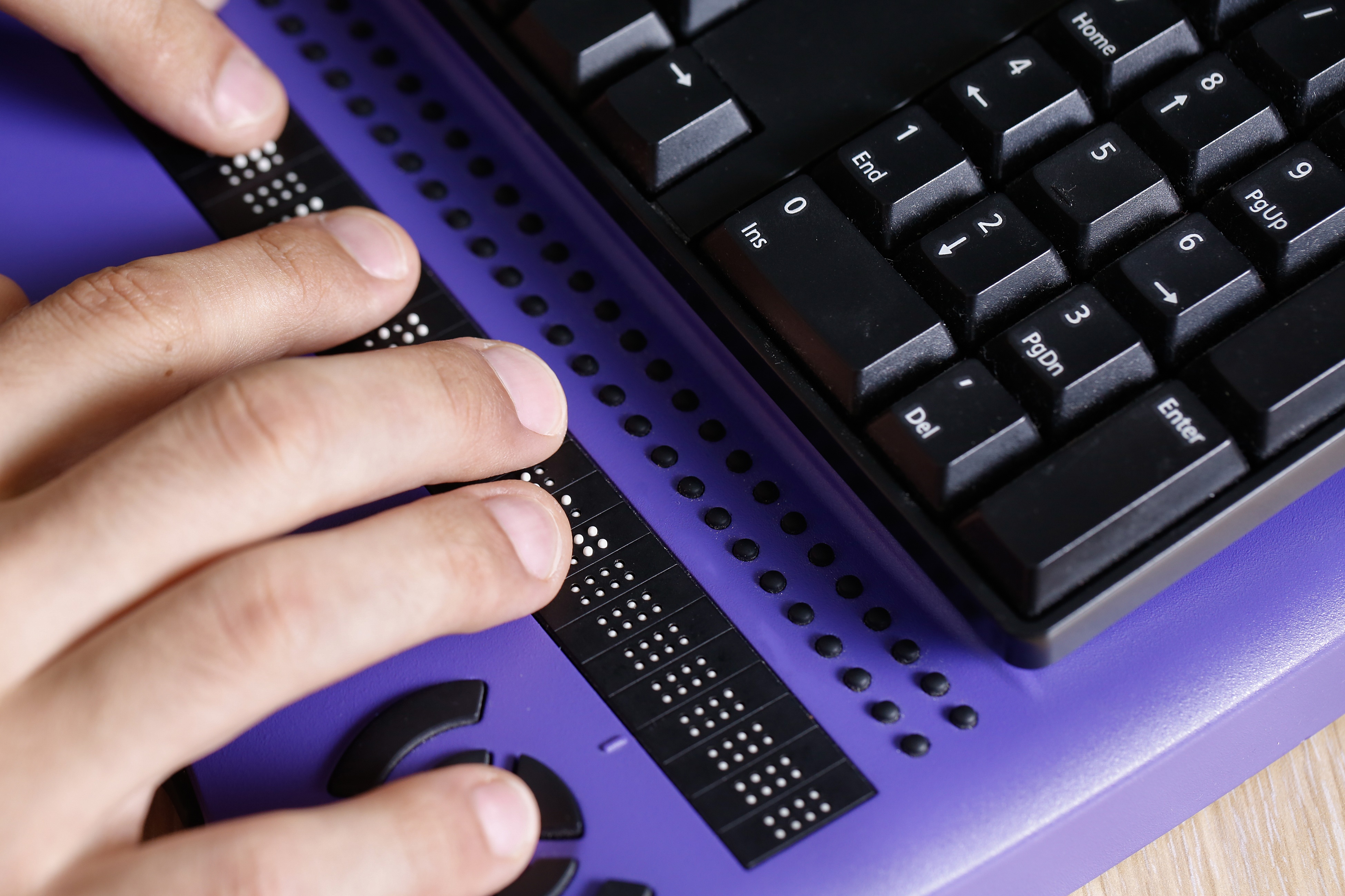The image depicts a white hand with short fingernails interacting with a Braille device positioned below a black keyboard. The person's fingers are gliding over the device, which features two rows of 2x4 grids containing small dots. These white dots, which can raise and lower, are arranged within black rectangles, providing tactile feedback for the visually impaired to read text from the screen. Above the Braille device, the black keyboard features keys labeled with numbers from 0 to 9 and various function keys such as insert, delete, and page down. The setup, which includes a purple base for the Braille device, showcases an ingenious method for enabling blind individuals to navigate and interact with computer content.